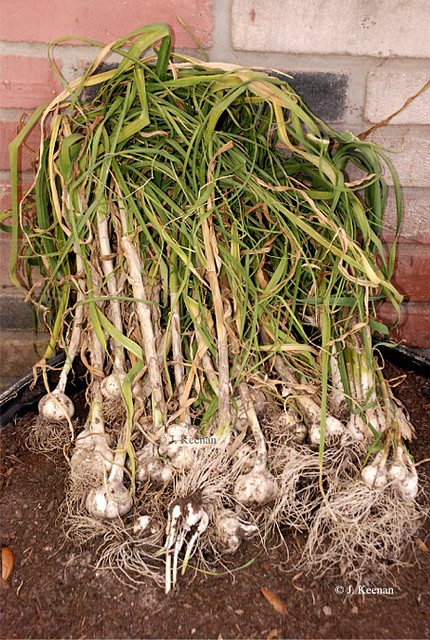This outdoor photograph captures an abundant harvest of what appears to be around 20 to 30 pieces of green garlic, freshly pulled from the soil. The garlic, with its long green stems and white bulbs still attached to the roots, is neatly arranged on top of a circular black planter. The rich, loose soil from the planter clings to the roots, emphasizing their recent extraction. The backdrop features a vibrant, multi-colored brick wall with shades of pink, red, orange, black, and white. In the bottom right corner, a watermark with the photographer's name, J. Keenan, is visible, marking the image's authenticity.